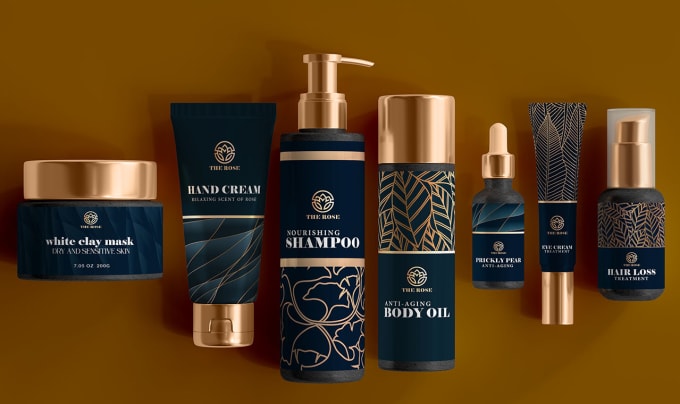The image depicts a neatly arranged assortment of seven toiletry items positioned horizontally against a dark brown background. Each product is contained within a black bottle adorned with intricate gold designs and gold lids, exuding a luxurious aesthetic. From left to right, the items include:

1. A round container of white clay mask with a smooth gold lid.
2. A hand cream in a sleek squeeze tube, also with a gold cap.
3. A pump bottle of nourishing shampoo featuring elegant gold lines and a scroll design on the bottom half.
4. An anti-aging body oil encased in a bottle decorated with delicate gold leaves.
5. A prickly pear serum, identifiable by its dropper cap.
6. An eye cream in a squeeze bottle capped with gold leaves.
7. A hair loss treatment with a pump covered by a plastic cap.

The cohesive branding across these items, likely labeled “The Rose," emphasizes a unified and premium brand identity.